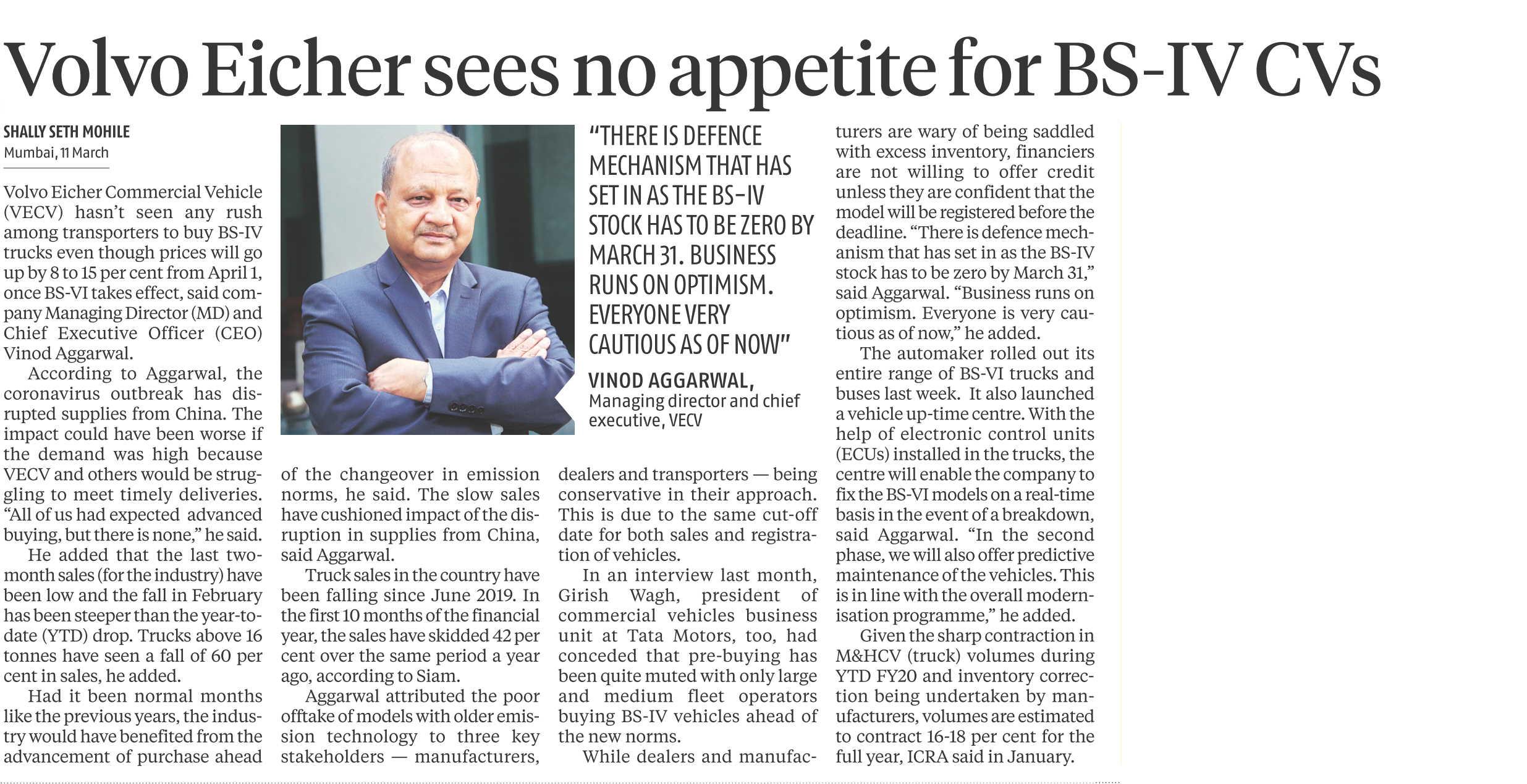The image is a detailed screenshot of an article from a newspaper, resembling a traditional print format. At the top, the headline reads, "Volvo Executive Sees No Appetite for BS IV Vehicles," with the title in bold, indicating a focus on current automotive industry trends.

On the left side, directly beneath the word "Volvo," there is a partial header that appears to read "Shally Says No Heel Mumbai Think Tank," possibly indicating the author or a related commentary.

Prominently featured in the center of the article is a photograph of a man dressed in a blue suit, standing with his arms crossed in front of his chest. This image is strategically placed between parts of the headline, specifically between "etch here" and "sees."

Below the words "no" and "appetite," a notable quote is displayed: "There is a defense mechanism that has set in as the BS IV stock has to be zero by March 31st." This statement suggests urgency in the context of regulatory compliance and the phasing out of BS IV vehicles.

Additionally, the article includes a subheadline or tagline, "Business World on Optimism," hinting at a broader theme of positive outlooks within the business sector despite challenges.